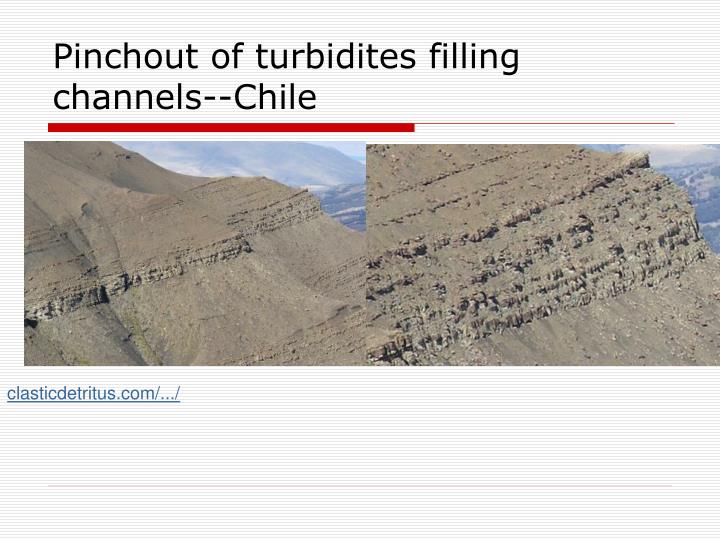The image depicts a large, hilly, open area, specifically the side of a brown hill or mountain, presumably located in Chile. The main focus of the image is on geological features, identified as "pinch out of turbidites filling channels." Turbidites appear as tracks or ridges on the slope, indicating various sediment layers accumulated over potentially thousands of years. The image is divided into two sections: the left half is a broader view, while the right half offers a closer, zoomed-in perspective. The background includes additional mountainous features, enhancing the sense of landscape depth. The caption at the top reads, "Pinch out of turbidites filling channels, Chile." At the bottom left and right corners, there is a URL: "clasticdetritus.com."